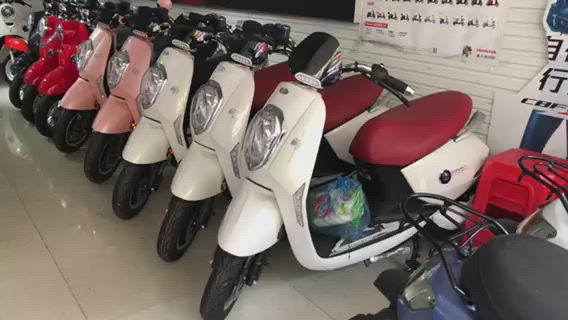The image likely captures a showroom in Asia dedicated to selling mopeds and scooters. The floor, covered in shiny white marble tiles, enhances the indoor setting. The main focus is a lineup of nine mopeds in various colors: three white, two pink, two red, and one black. Some of the scooters have tied-on black helmets and bags, and they seem designed for one to two passengers. In the background, there are posters and a TV with Asian characters, suggesting the location is in an Asian country. Additionally, two mopeds face away from the camera, showing the areas where backpacks can be tied down. A little red stool is also placed among the scooters, and there are two visible four-wheelers on the right side. The detailed display, including a cutout poster, suggests this showroom offers a wide range of motorized vehicles.